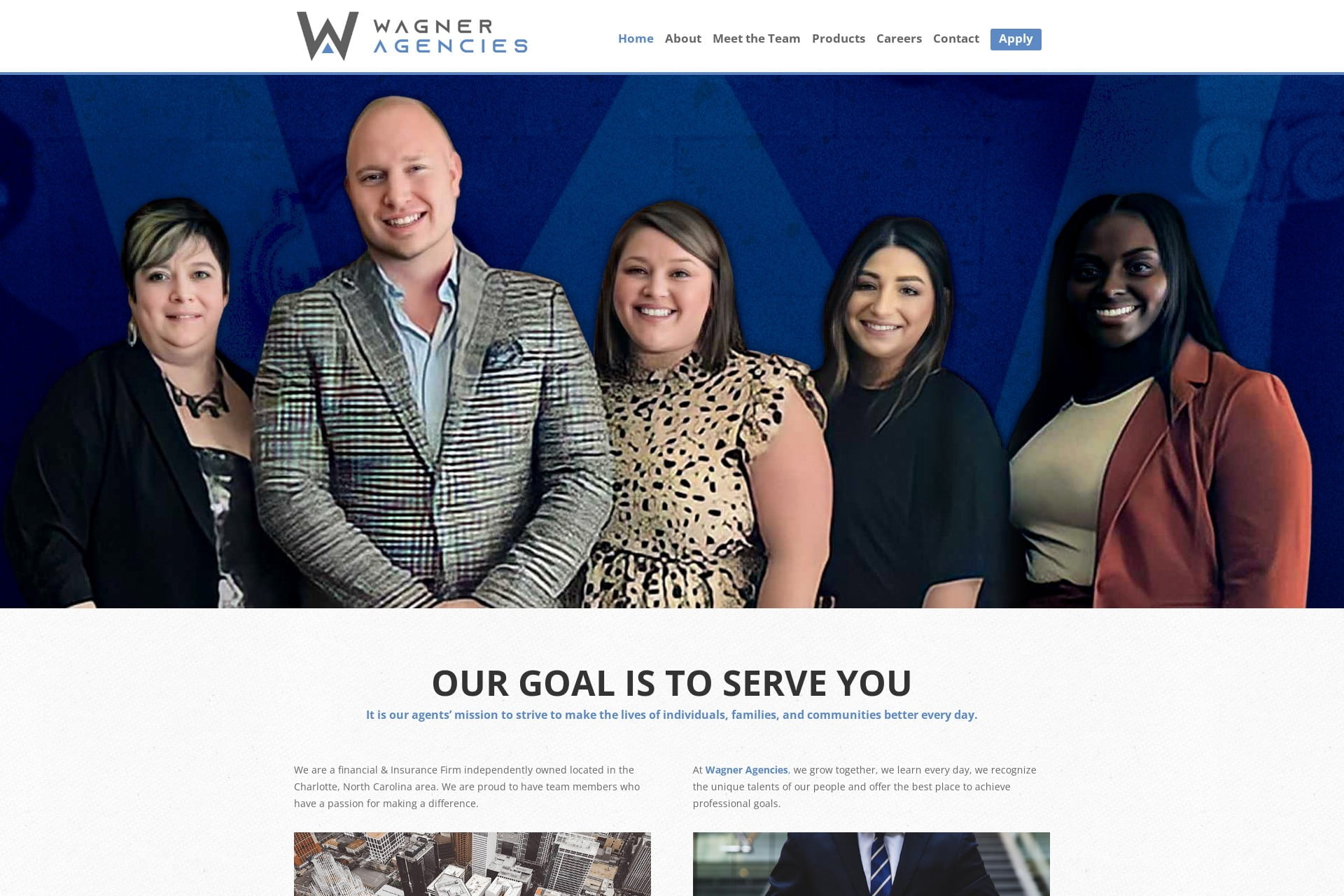The webpage features the Wagner Agencies logo prominently at the top left corner. The logo comprises a stylized "W" and the text "Wagner Agencies." On the top right, a series of navigation tabs facilitate easy access to various sections of the site. The tabs are labeled from left to right as follows: Home, About, Meet the Team, Products, Career, Contact, and Apply.

Below the navigation bar is a group photograph of five individuals who are all looking directly at the camera and smiling. The group consists of one man and four women. 

- The woman on the far left has a distinctive hairstyle with black and blonde hair. Her facial features, including her eyes, ears, nose, and mouth, are clearly visible. She is wearing a round, black earring in her right ear and a black necklace. Her outer garment is a black sweater.

- Next to her stands a bald man, also smiling. His eyes are visible, and he is dressed in a grey jacket paired with a light blue shirt underneath.

Below the image, a mission statement reads, "Our Goal is to Serve You. It is our agent's mission to strive to make the lives of individuals, families, and communities better every day." 

To the left of this statement, there is an additional message that states, "We are a financial insurance firm, independently owned and operated."